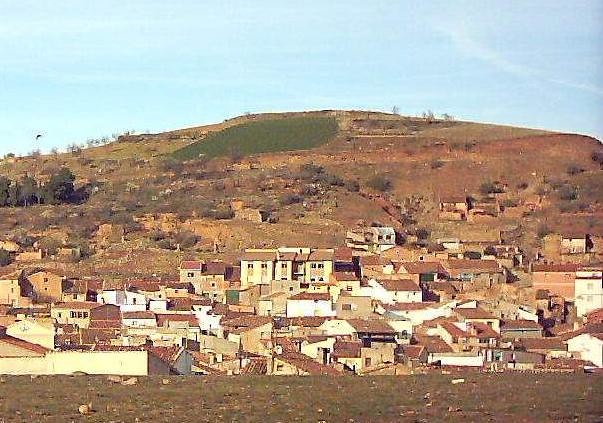This photograph captures a small, older town nestled at the base of a gently sloping hill. The buildings are closely packed, with yellow-white walls and predominantly medium to dark brown roofs, some appearing worn and aged. In the foreground, sparse trees and possibly small mammals or rocks dot the grassy terrain. The town's structures vary in height, with a few two to three-story buildings centrally located among predominantly single-story houses. The background is dominated by the hill, which transitions from sparsely placed homes and brownish-brick buildings to patches of grass and scattered trees as it rises. The sky above is a clear, light blue with a few wispy clouds, providing a serene backdrop to the quaint, rustic scene.